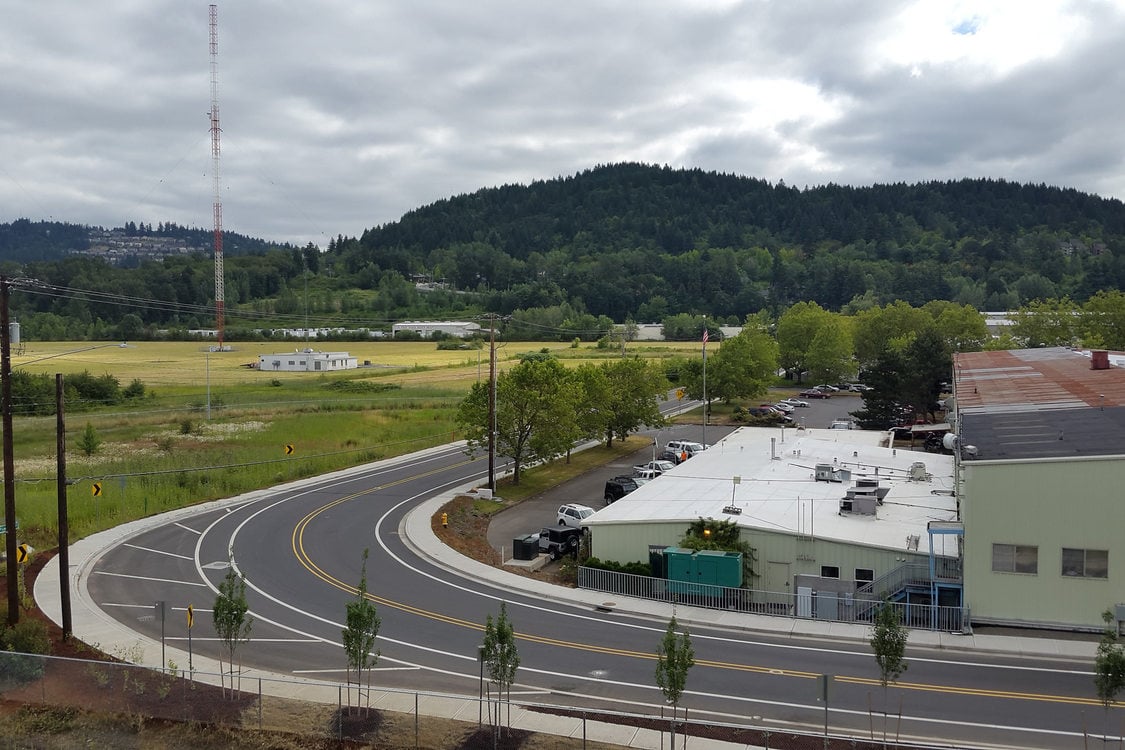The photograph, taken outdoors during the daytime, captures a panoramic view of a rural town with a two-lane paved road that begins in the lower right-hand corner, extends towards the left side, and then sharply turns at a 90-degree angle up towards the center, disappearing behind some foliage. The road features a solid double yellow line down the middle and white lines on either side, with a wide apron for parking. Yellow signs with black arrows signal the approaching turn. Bordering the road at the bottom, a chain-link fence encloses a walkway area dotted with sapling trees.

On the right-hand side of the road, we see a commercial complex featuring two flat-roofed buildings. The first building, which sits at road level, is clad in light mint green siding and has an orange and gray roof, while the second building, slightly sunken below road level by the parking lot, has the same siding but with a white roof. Several cars are parked in the lot, bordered by trees and sidewalks. A row of cars is also parked in front of the larger, single-story building, which features a two-story section with a visible fire escape and windows.

On the left-hand side of the road's bend, a grassy field sits alongside a few houses, while in the background, hills covered in dark green trees rise up beneath a gray, cloudy sky. A radio aerial can be seen jutting up from the treeline on one of the hills. This tranquil, rural scene combines natural beauty with signs of small-town life.